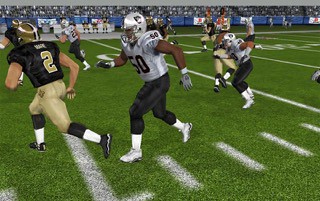This small horizontal photograph captures a dynamic action shot of an American football game on a pristine grass field marked with crisp white yard lines. The scene features two teams in mid-play: the defensive team, clad in silver-white jerseys, silver-white helmets, navy blue pants, and white cleats, and the offensive team, distinguished by navy jerseys, gold pants, navy and white socks, black cleats, and gold helmets. At the center of the action, an offensive player, who is Caucasian, can be seen running with the football, pursued by several defensive players. Among the visible defensive players, two are African-American and one is Caucasian. In the background, the stands are partially visible along with people standing on the sidelines, adding to the atmosphere of the game.